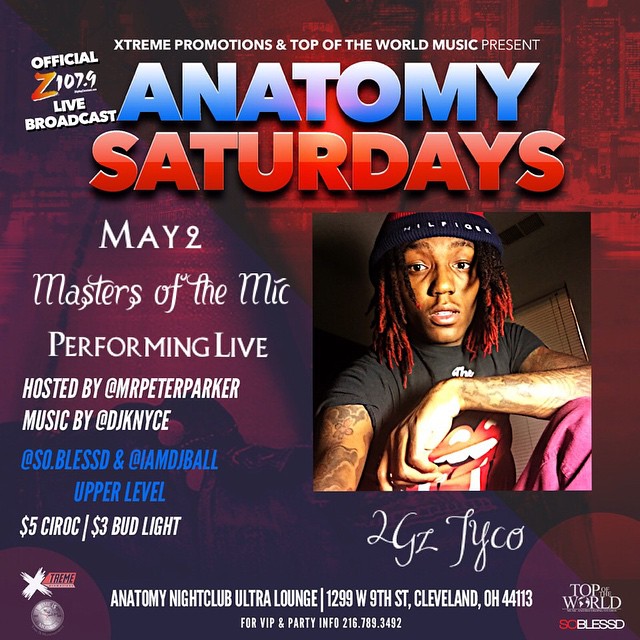This advertisement flyer promotes a musical event at Anatomy Nightclub Ultra Lounge, located at 1299 West 9th Street, Cleveland, Ohio, 44113. The event, titled "Anatomy Saturdays," is presented by Extreme Promotions and Top of the World Music, with an official Z107.9 live broadcast. The event is set for May 2nd and features "Masters of the Mic Performing Live," hosted by Mr. Peter Parker, with music by DJs including DJ Nice, So Blessed, and DJ Ball on the upper level. The flyer also highlights drink specials: $5 for Ciroc and $3 for Bud Light.

Central to the flyer is a striking image of an artist identified as YGZ Tycho. He is a black man with long, black and red dreadlocks, wearing a red and black Tommy Hilfiger beanie. He is dressed in a black Rolling Stones t-shirt featuring a prominent mouth and tongue graphic, and red jeans. The lower sections of the flyer feature branding and contact information for VIP and party details, including a phone number: 216-789-3492. The background of the flyer is predominantly red with some purple elements, adding to its vibrant, eye-catching design.